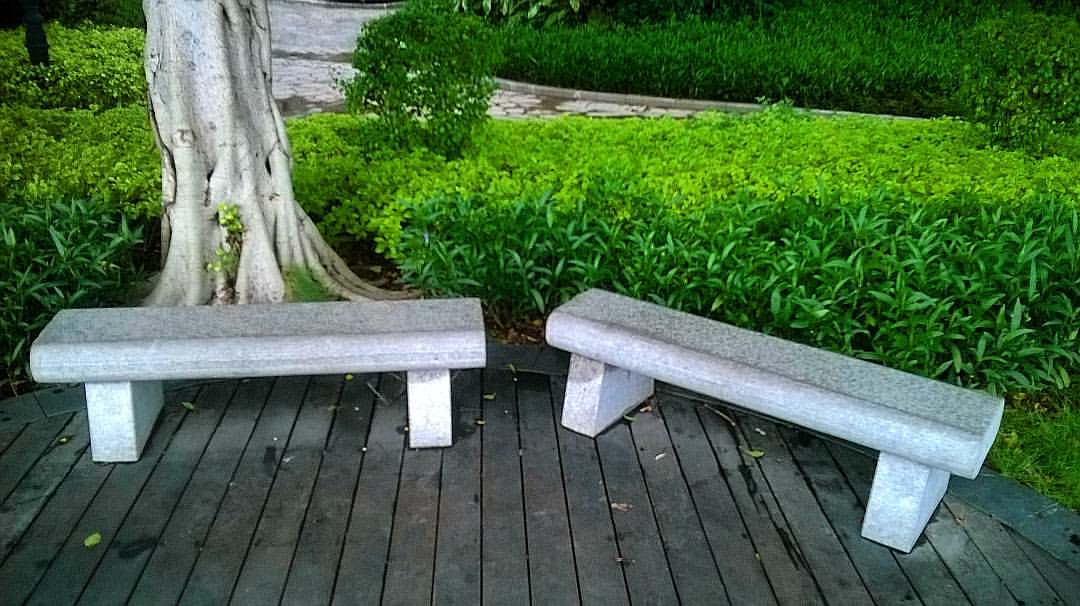This photograph captures a serene outdoor garden scene featuring a dark gray, wooden deck with two slightly weathered white cement benches. The benches are rectangular and supported by cement blocks, positioned prominently at the front. Behind the left bench, a striking white tree trunk stands out, partially visible and surrounded by lush, vibrant green hedges and bushes of varying heights and shades. Beyond the greenery, a body of water, possibly a pond or river, is lined with a concrete embankment. The various greens of the shrubbery create a rich, textured backdrop for the scene, with some having small, short leaves and others boasting longer foliage. The overall image is a harmonious blend of natural and man-made elements, highlighting the peaceful integration of outdoor furniture and lush plant life.